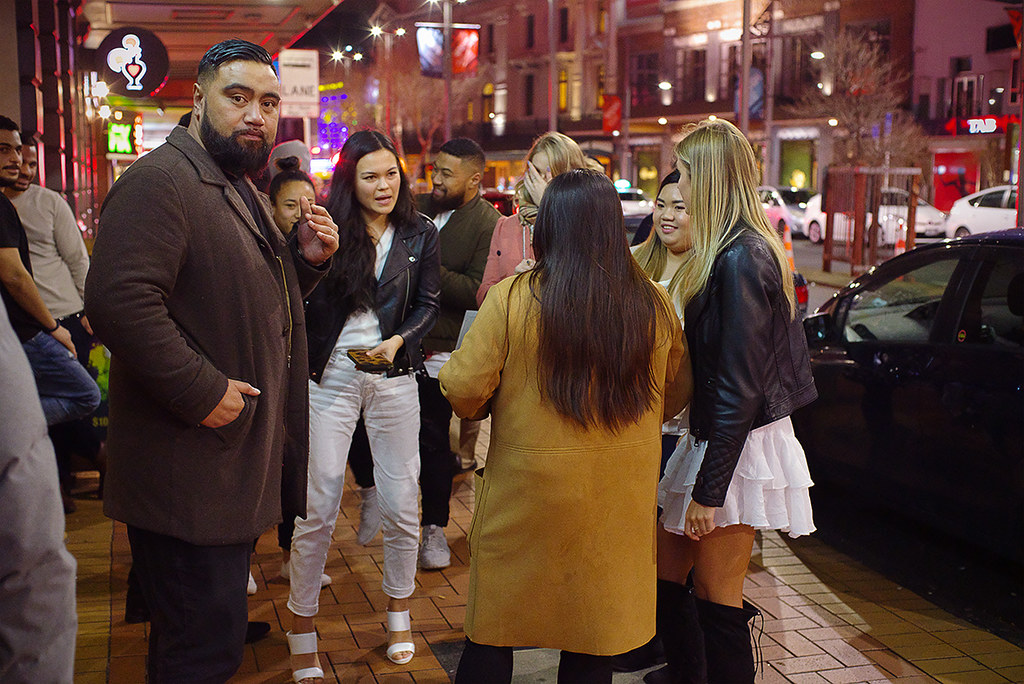In this nighttime city scene, a lively group of well-dressed people gathers on a neon-lit sidewalk outside a bar, with a prominent martini glass sign hinting at the establishment. The focal point is a semi-circle of six women engaged in animated conversation, their attire ranging from leather and suede jackets to skirts and pants, all with carefully styled hair. To the left of the group, a man with a brown jacket, black pants, and a neatly styled back hair and black beard stands with his body facing the women but his head turned to stare directly at the camera with an expressionless gaze. His hand rests casually in his pocket. The bustling backdrop features parked cars and additional pedestrians milling about, contributing to the vibrant nightlife atmosphere filled with colorful neon lights from various bars lining the street.